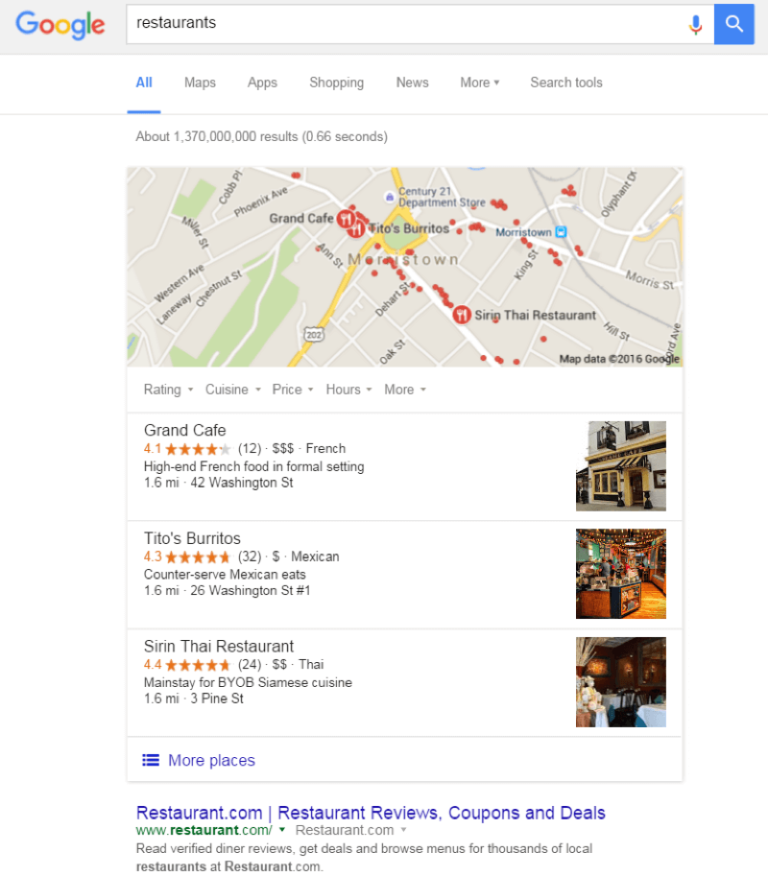**Image Description: Google Search Results for Restaurants**

The image captures a Google search page specifically for restaurants. At the top, you can see the title bar and the search bar directly below it. Beneath the search bar, there are several navigational tabs labeled "All," "Maps," "Apps," "Shopping," "News," "More," and "Search tools."

Following these tabs, the image shows a large street map peppered with red dots indicating various restaurant locations. Additionally, three larger circles feature fork and knife icons, representing key dining establishments. The search results are filtered by rating, cuisine, price, hours, and more.

The first restaurant listed is the "Grand Cafe," known for its high-end French cuisine served in a formal setting. There is a small, square photo of the building's facade on the right side.

The second listing is "Tito's Burritos," accompanied by a picture of the restaurant's interior.

The third listing is a "Sentai Restaurant," with an interior photo as well.

Below these primary entries, there's a link labeled "More places" to explore additional restaurants.

At the very bottom of the page, there's a snippet from restaurant.com offering restaurant reviews, coupons, and deals. It invites users to read verified diner reviews, get deals, and browse menus for thousands of local restaurants.